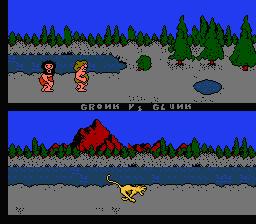This digital artwork is split into two distinct sections. The upper portion depicts two figures resembling cavemen standing beside a serene, blue lake. The figure on the left sports dark hair and a red outfit, while the one on the right has blonde hair and is dressed in yellow. Adjacent to this lake is a smaller, circular blue pond. The surrounding landscape features gray ground and a ring of lush, green trees with brown trunks, including pine trees in the background and to the right. Above, the sky is a clear, vivid blue.

Separating the two scenes is some text. The lower portion of the image illustrates a long, narrow lake stretching horizontally across the frame. Here too, the ground is gray. In the center of this section, a yellow animal dashes across the land. The backdrop includes a bright blue sky, dense green trees, and a striking red mountain, adding depth and vibrancy to the scene.